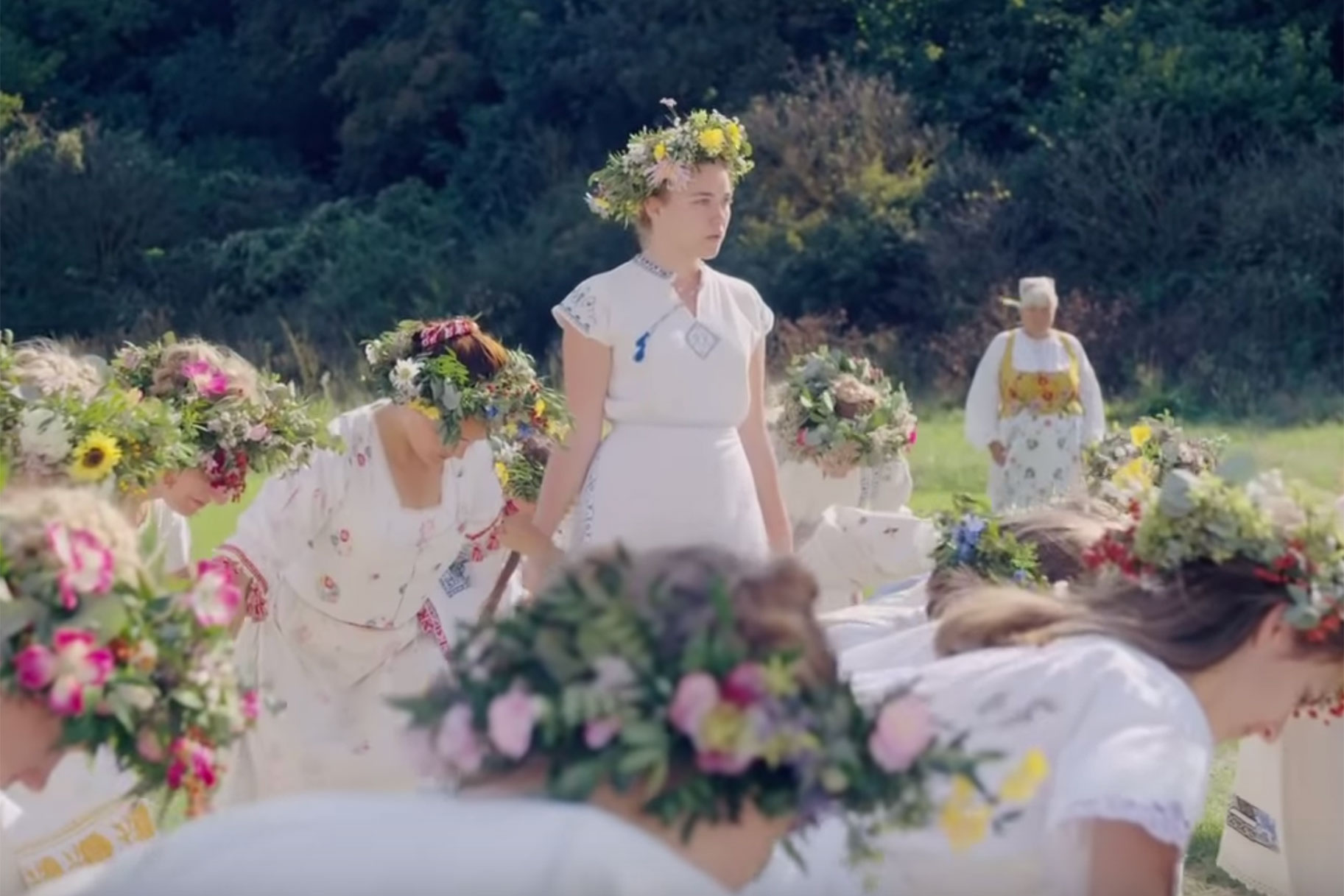The image depicts an outdoor scene, possibly from a movie, featuring a group of seven or eight women dressed in white dresses adorned with floral crowns. They are in a grassy area and most of them are kneeling or bending over, suggesting some form of focused activity. One woman stands in the middle of the group, distinctive with her floral crown and white dress, commanding attention. In the background, lush green trees and bushes frame the scene, adding a natural, serene backdrop. An older woman, noticeably different in attire with a white dress and a yellow apron instead of a floral crown, stands apart, observing the others with a head wrap on. The overall scene appears slightly hazy, adding a dreamy or ethereal quality to the image.